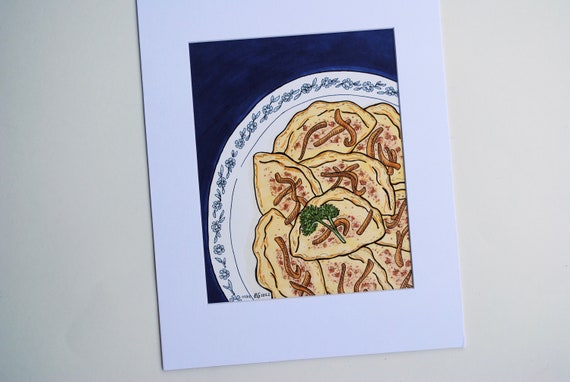This is a detailed color photograph depicting the front cover of a greeting card. The centerpiece of the card features a white plate adorned with a delicate gray floral border around its edges and an inner thin blue line. Placed elegantly on this plate are beige, crimped raviolis, each forming a half-circle shape with bumpy ridges on top. The raviolis are garnished with orange-tinted fried onions and a fresh green sprig of parsley resting atop one of them. The plate is set against a rich navy blue background, giving a striking contrast to its contents. This image is framed by a large white border, creating a clean and organized presentation on what appears to be either a white canvas or a piece of paper resting on an off-white surface, slightly tilted to the left at the top.